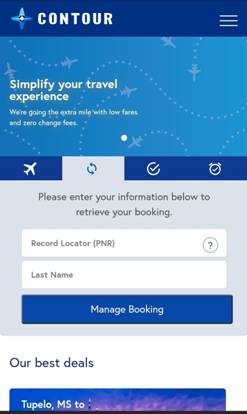The image appears to be a screenshot taken on a mobile device. At the top of the screen, there is a dark blue banner featuring a star icon on the left, followed by the word "Contour" in bold white text. On the far right of the banner, there are three horizontal lines indicating a menu.

Below the banner, a light blue background encompasses a rectangular area filled with airplane icons followed by trailing dots, suggesting flight paths. In the bottom left corner of this area, white text reads: "Simplify your travel experience. We're going the extra mile with low fares and zero change fees."

Directly beneath this, a small blue border separates the light blue section from various symbols: an airplane, two arrows forming a circular pattern (one pointing left and one pointing right), a circle with a checkmark, and a clock. The arrows, which indicate a change option, seem to be selected by the user.

Further down, a gray box contains a prompt that says, "Please enter your information below to retrieve your booking." Within the box are two rectangular input fields: one labeled "Record Locator PNR" with a question mark icon beside it, and the other labeled "Last Name." Beneath these fields, a blue button labeled "Manage Booking" invites the user to proceed.